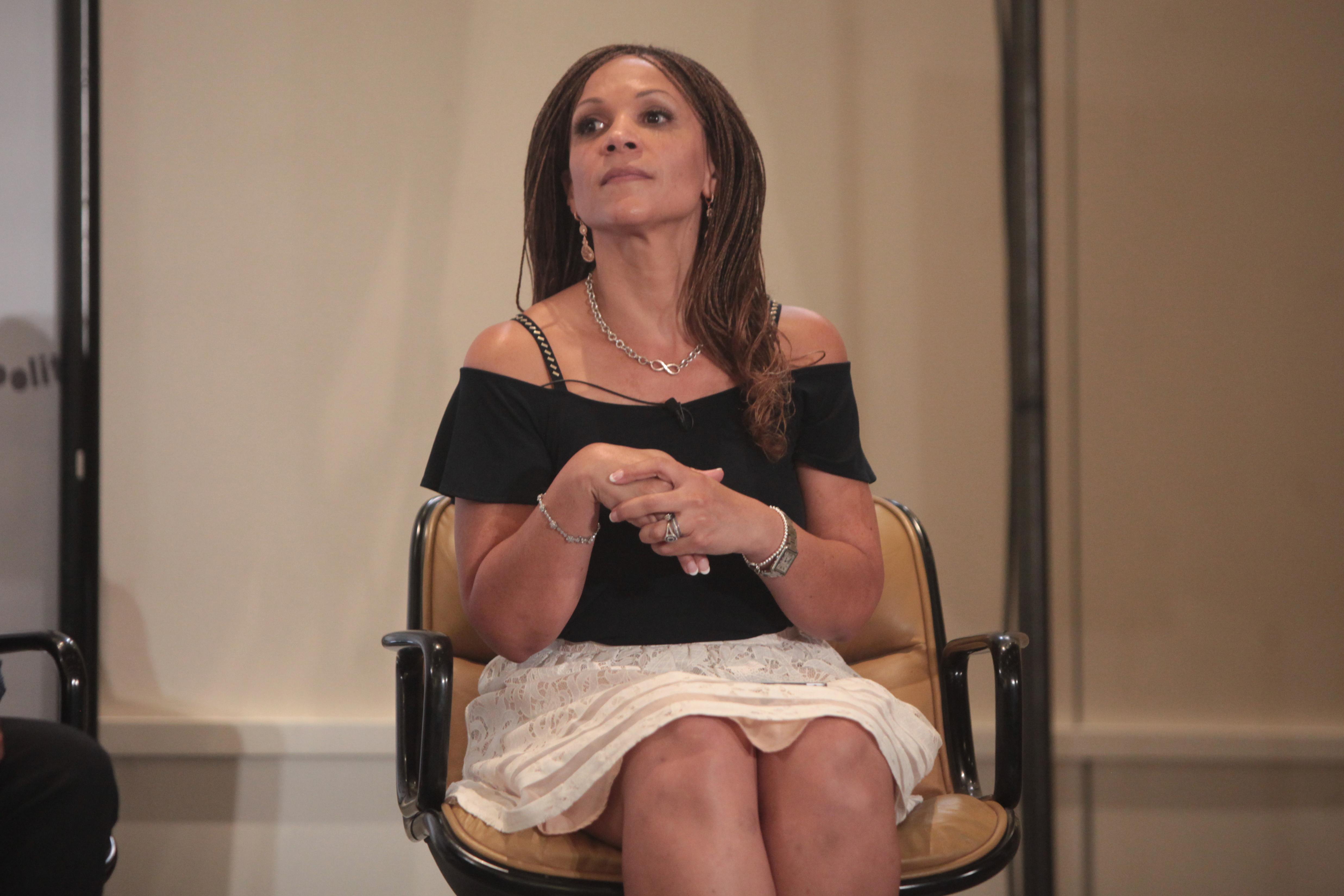In this image, a light-skinned, middle-aged woman is seated at the center, looking slightly upwards and to her right. She has long brown hair and is adorned with a variety of jewelry, including a silver necklace, bracelets, watches, and rings. She wears a black top that reveals her shoulders and a white or beige skirt. The chair she occupies features a light orange or beige cushion with shiny metal or black railings. Another chair is positioned next to her on her right. The background is stark with mostly blank walls in off-white or beige shades and vertical black bars. Her hands are held together in front of her chest. The setting appears to be some event where someone might be speaking, indicated by the simplicity of the surroundings and the focus on the seated woman. A text overlay in the image indicates "there is no sex in this picture." The colors in the scene include beige, tan, brown, white, and black.